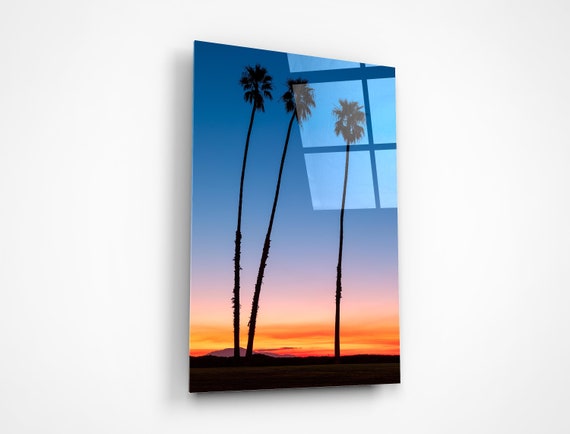The image depicts a glossy, laminated poster on a white wall, reflecting the light pattern from a window on its right side. The poster features a beach scene during sunset, with three tall palm trees extending upwards from a dimly lit, sandy ground. The two trees on the left lean slightly towards each other while the tree on the right stands apart. The sky transitions from a dark blue at the top to warm hues of orange, red, and pink near the horizon, indicating the setting sun. The overall ambiance of the picture is serene, characterized by the silhouetted palm trees against the colorful twilight sky.